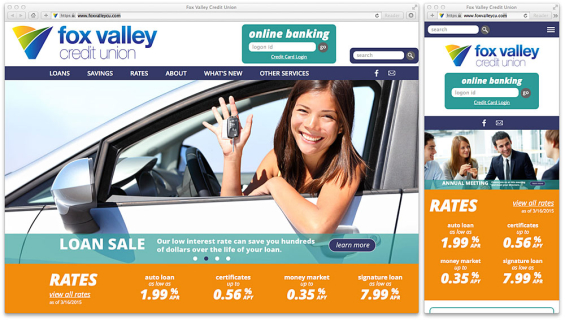The image depicts the homepage of the Fox Valley Credit Union website. At the very top, a gray background hosts the URL. Just beneath the URL, there's a prominent logo starting from the top left, shaped like a "V" with sections colored yellow, green, and blue. The text "Fox Valley" appears in blue, and "Credit Union" is displayed in a smaller, blue line style.

To the right, there is a turquoise-colored square labeled "Online Banking," which includes a mini search bar and a black "Go" button. Further right, there is another mini search bar.

Below this top section, the webpage displays six categories in small white text. Directly underneath, an image shows a smiling woman in a car, holding a car key with one elbow resting out the window. The car is a mix of turquoise and silver or white, set against a light blue upper background.

The section below this image includes the text "Loan Sale" presented in white, followed by "Rates," which lists four rate figures: 1.99%, 0.56%, 0.35%, and 7.99%.

Adjacent to this section, on the right side, there is a minimized version of the main screen, but it features a group of people instead of the woman in the car.